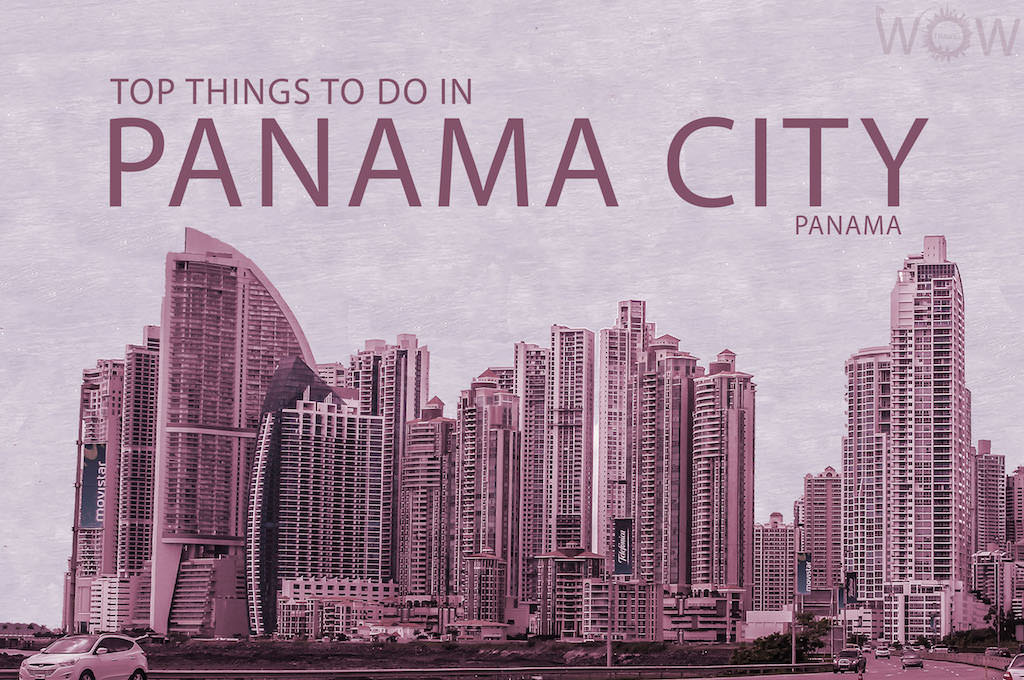The image features a captivating, futuristic skyline that immediately catches the eye with its towering, aesthetically pleasing buildings. These skyscrapers, some appearing to be at least 50 stories high, dominate the scene with their sleek architectural designs, all bathed in a harmonious purple and violet hue. The background accentuates this color palette with a soft, almost ethereal white that transitions seamlessly into the purple tones, suggesting the application of a visual filter that enhances the overall allure.

At the bottom, a serene three-lane highway stretches horizontally across the image. It is lightly trafficked, with only a few cars dispersed along its length, lending a sense of calm and quiet. The highway is punctuated at intervals of approximately 20 to 30 feet by banners, though the content on these remains unreadable, adding an element of intrigue. A sparse scattering of trees lines the lower edge of the image, providing a subtle natural contrast to the urban landscape.

Across the top of the image, in moderately sized text, the phrase "Top Things to Do in" is displayed, leading into the focal point of the ad - the bold, large, purple title "Panama City." The geographic identification is completed with the word "Panama" in smaller text positioned in the bottom right corner. This visually striking and well-composed advertisement effectively conveys a sense of modern elegance and tranquility, making Panama City a compelling destination for potential visitors.